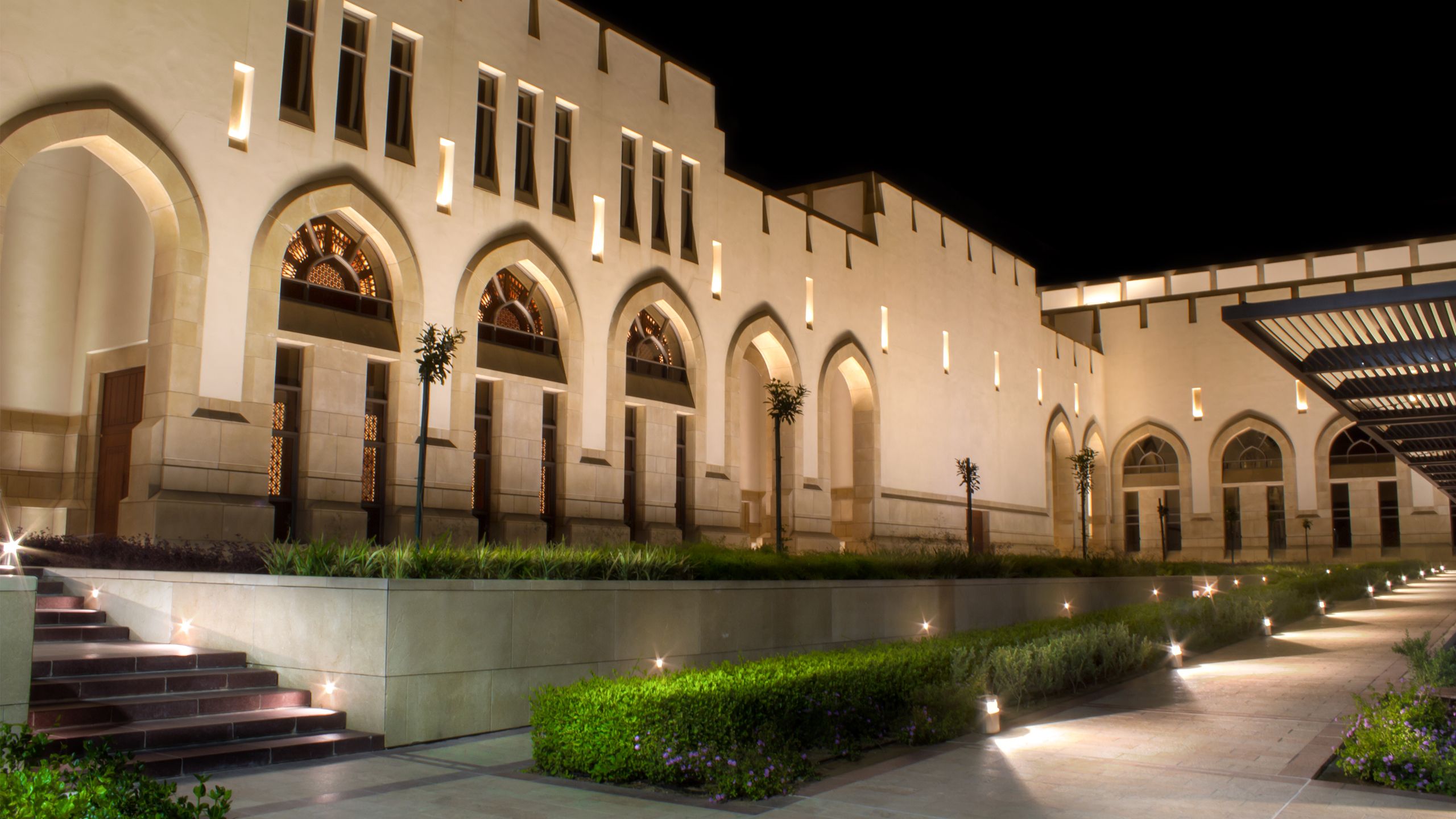A photo taken at night captures the exterior of a large, ornate building with a castle-like appearance and a somewhat Arab architectural influence. The building stands out against the pure black sky due to the various lights illuminating its features. It is at least two stories tall with a series of pointed archways, each containing brown rectangular doors, and a row of metal-grated windows above. Additionally, there are three sets of three long windows that appear dark in the image. While the building's walls have a pinkish hue under the artificial light, they might be white or a brownish-tan color.

In front of the building, a well-made concrete or stone walkway leads up to a staircase on the left, made of red bricks, and a ramped walkway on the right, adorned with short hedges. Elevated sections of the property feature more bushes and trees, adding greenery to the scene. The area is well-lit with canister lights and embedded wall lights, highlighting the stairway and a marble wall, providing a striking contrast to the dark sky. The overall scene is well-composed with an emphasis on the intricate details of the building's structure and the careful placement of lighting, which accentuates the building's design and the surrounding landscaping.